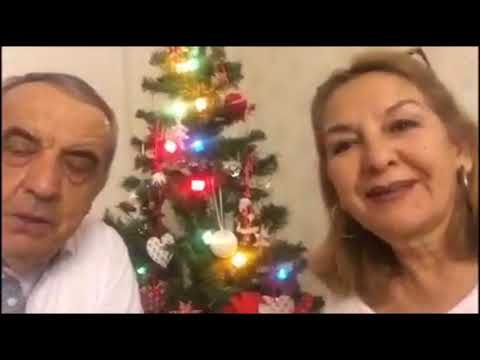The image, a horizontally aligned rectangular photograph with thick black borders at the top and bottom, features an elderly couple flanking a Christmas tree adorned with colorful ornaments and lights, including red, blue, and yellow. The man, appearing on the left, has a receding hairline with combed-over brownish-gray hair, dark eyebrows, and bags under his eyes. His thin lips are slightly parted, and his eyes are closed, likely caught mid-blink. Dressed in a white button-down collared shirt, he is partly cut off by the image's edge. To the right stands the woman, smiling at the camera with her lips slightly parted and wearing dark lipstick. Her shoulder-length brown hair is accented by large hoop earrings and glasses propped atop her head. She is wearing a white blouse. Both individuals appear to be in their 60s or 70s. The background is a beige, tan-colored wall, and the image captures them from their chest up in what seems to be an indoor setting, possibly someone's home.